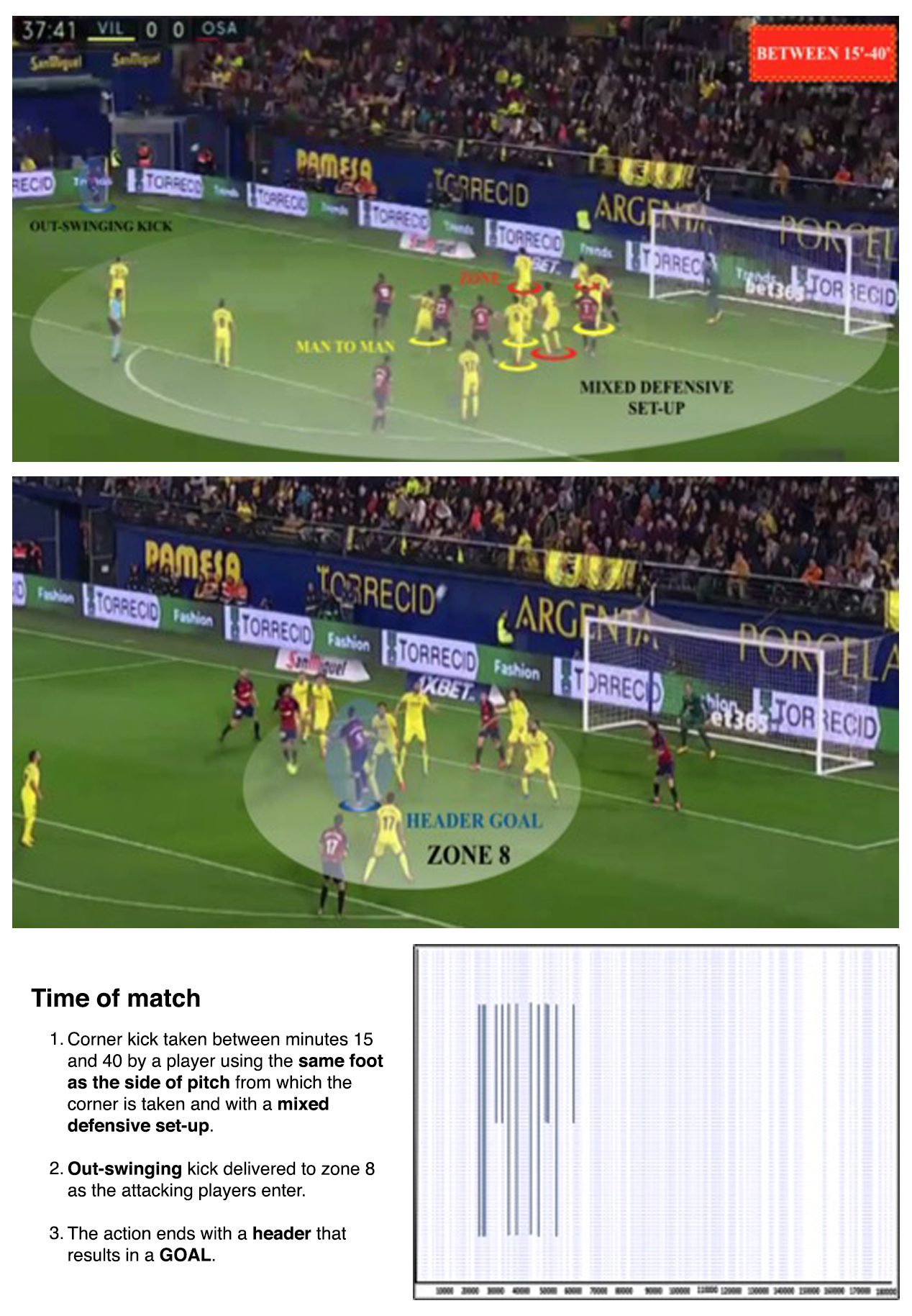The image is a detailed graphical illustration or AI-generated depiction of a soccer match with a focus on corner kick strategies. The top of the image contains text stating "between 15 and 40 feet." The bottom has comprehensive captions explaining a three-step process called "time of match," which details how to execute and benefit from a corner kick. 

The first step describes the setup: "Corner kick taken between minutes 15 and 40 by a player using the same foot as the side of the pitch from which the corner is taken, with a mixed offensive setup." The second step shows "Out swinging kick delivered to zone 8 as the attacking players enter." The third and final step illustrates "The action ends with a header that results in a goal."

The image itself portrays players in yellow and red jerseys positioned according to these steps on different sections of the soccer field. The top portion of the image focuses on the mixed offensive setup, while the bottom highlights the header goal in zone 8, featuring a circular focus highlighter around the players involved. The scene is set in a soccer stadium with sponsorship banners that include references to Argentina and Torres Seed, adding authenticity to the match setting. Key terms such as "same foot as the side of the pitch," "mixed defensive setup," "out swinging kick," "header," and "goal" are emphasized in bold to guide the viewer through the tactical explanation.